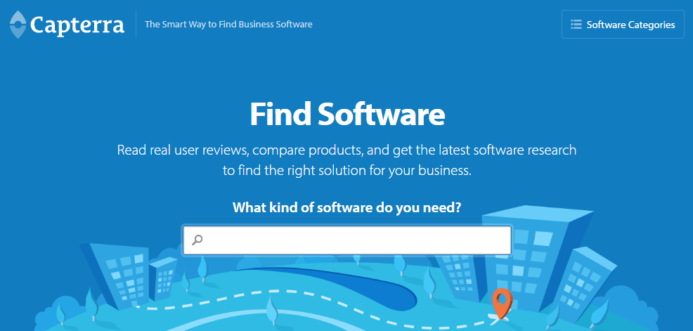The webpage for Camtira, a platform dedicated to helping users find business software, features a clean and modern design. In the upper left corner, the company's name and tagline, "Camtira, the smart way to find business software," are prominently displayed. On the upper right, a menu icon suggests additional navigational options.

Just below the main header, a button labeled "Software Categories" offers quick access to various types of software. The centerpiece of the page is a bold headline that reads "Find Software" in large, white letters. Directly underneath, a subheading encourages users to "Read real user reviews, compare products, and get the latest software research to find the right solution for your business." 

A more prominent prompt in slightly bolder white text asks, "What kind of software do you need?" This is followed by a search box with a magnifying glass icon, facilitating easy and intuitive searching.

The background image provides a touch of visual interest, featuring a stylized cityscape with vector graphics of buildings and trees. A road runs through the scene, marked by a dotted white line. There's an artistic element with an oval shape in an orangish-reddish hue, partially transparent, allowing glimpses of the background cityscape. The horizon curves gently from left to right, creating a dynamic backdrop. The sky, rendered in a light teal-blue color, enhances the overall modern and tech-savvy aesthetic of the webpage.